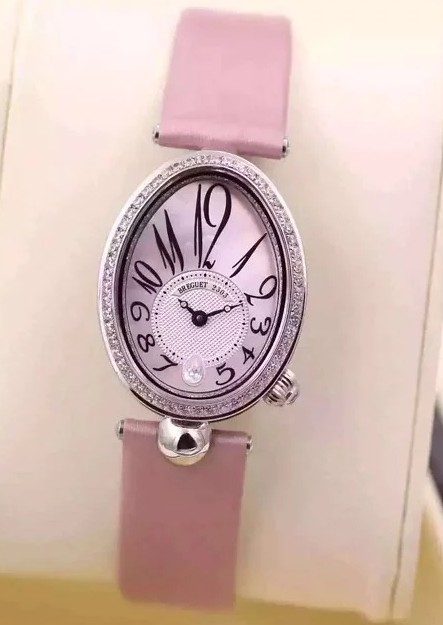Close-up photo of an elegant wristwatch resting on its display case. The watch features an oval face adorned with a border of diamond studs, adding a touch of luxury and shimmer. The dial displays bold, exaggerated numbers, creating a striking and somewhat optical illusion-like effect. The number 12 is the largest, dominating the top of the watch face, while the numbers gradually decrease in size down to the 5. At the 6 o’clock position, instead of a numeral, there is a small white, crystal-like embellishment. Moving past it, the numbers begin to increase in size again, with the 7 through 11 progressively getting larger, leading back to the prominent 12. The watch straps are a soft pink hue, adding a delicate and feminine touch. The entire watch is placed on a white display stand, which itself rests on a khaki-colored surface. The close-up nature of the photo focuses solely on the watch, leaving little else visible in the background.